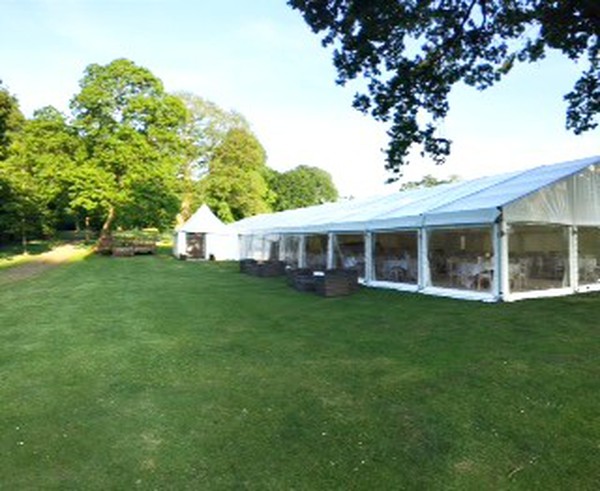The image showcases a picturesque garden setting with a large, white party tent positioned on the right side. The tent features a blue roof and white framework, and is set on a lush, green lawn that appears well-maintained. Inside the tent, numerous tables covered in white tablecloths and surrounded by white chairs are visible, suggesting it might be a venue for a wedding reception or similar event. Outside the tent, there are brown wooden tables and chairs arranged for additional seating. 

In the background, a cluster of tall, verdant trees can be seen, contributing to the serene atmosphere. These trees extend high into the sky, and there’s a smaller structure with a pointed, white, triangular roof behind the main tent, hinting at another entrance or exit. There is also a dirt road visible in the upper left corner, running under one of the large trees.

The sky is a light blue with some white patches, indicative of a clear midsummer day. In the upper right corner of the image, tree branches hang over the tent, adding a natural canopy effect to the scene. Overall, the image exudes a festive and inviting ambiance, perfect for an outdoor celebration.